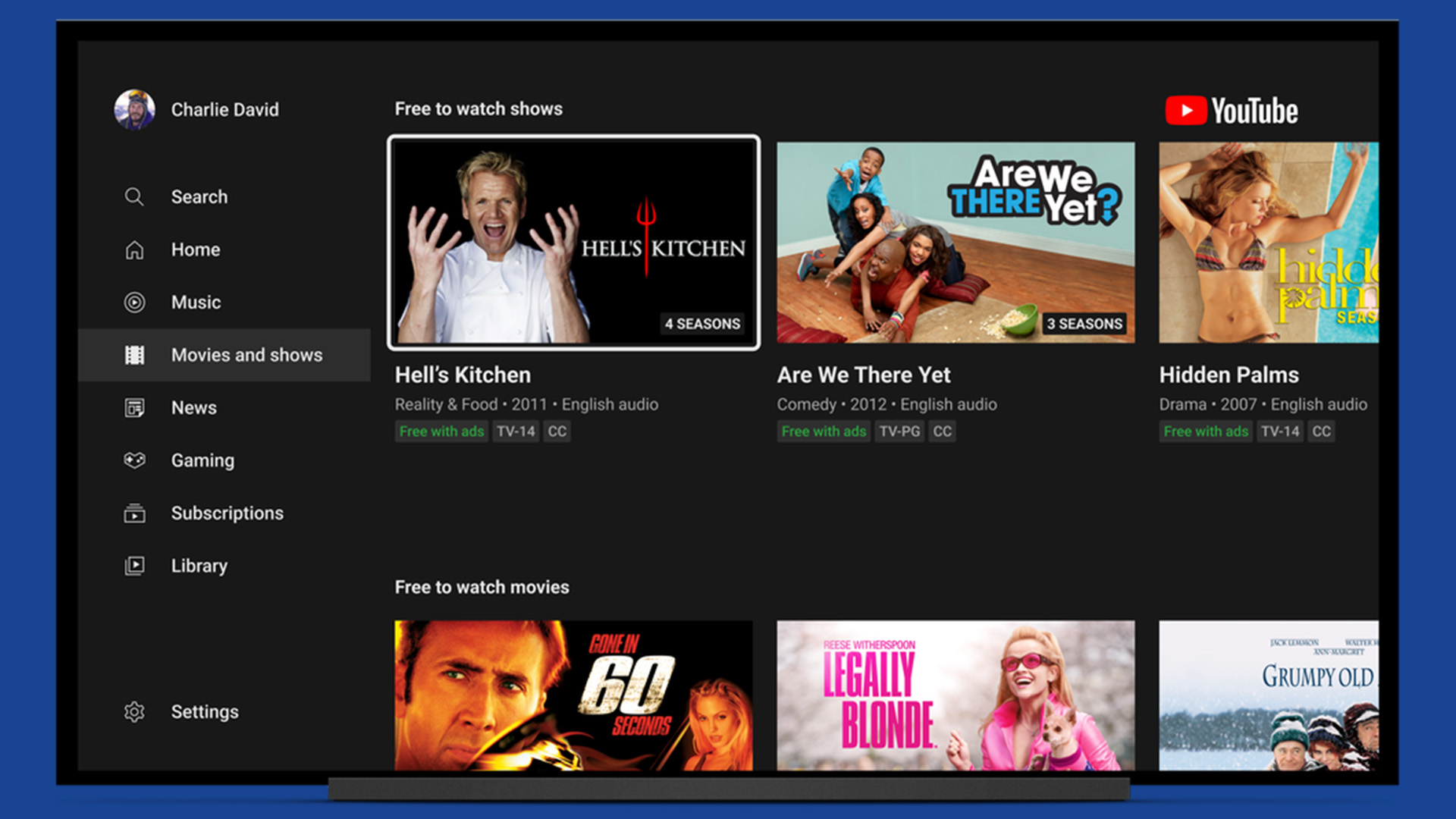The image depicts the YouTube app displayed in dark mode. The app interface is predominantly dark, providing a sleek and eye-friendly viewing experience. The account belongs to a user named Charlie David, whose profile picture features a man wearing a hat.

On the left side of the app, a vertical sidebar showcases various navigation tabs. These tabs, listed from top to bottom, include Search, Home, Music, Movies & Shows, News, Gaming, Subscriptions, and Library. Just below them is the Settings option.

The user is currently looking at the "Movies & Shows" section, indicated by the lighter color of the button. The section highlights a category labeled "Free to Watch Shows" at the top. Featured prominently are three popular titles: "Hell's Kitchen," "Are We There Yet?", and a movie called "Hidden Palms."

Beneath this, the section "Free to Watch Movies" is introduced, with titles such as "Gone in 60 Seconds," "Legally Blonde," and "Grumpy Old Men" available for viewing. The layout and contents clearly emphasize free entertainment options curated for the user.